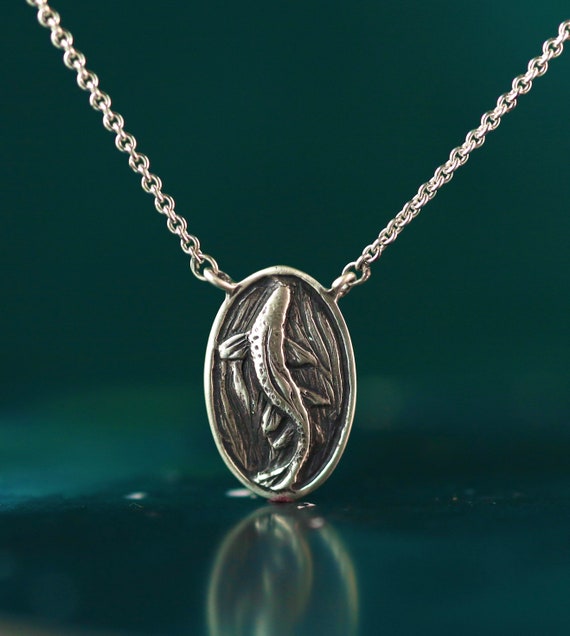This is a detailed close-up photograph of a well-polished silver necklace displayed on a dark green tabletop. The chain is elegantly suspended, extending to the top left and right, revealing a reflective and smooth surface that mirrors the necklace's intricate details. At the center of the silver chain hangs an oval-shaped pendant, featuring a meticulously carved fish. The fish appears to be viewed from above, with two fins on top, legs-like extensions at the bottom, and a long tail, possibly resembling marine creatures such as a shark, dolphin, or even an alligator. The fish's body is adorned with dot-like structures and is surrounded by wave-like engravings, suggesting it is swimming through the water. The pendant itself has a dark pewter or wooden appearance with black shading, contrasting beautifully with the silver chain. The professional lighting enhances the necklace's polished metal without causing any distracting reflections or highlights.